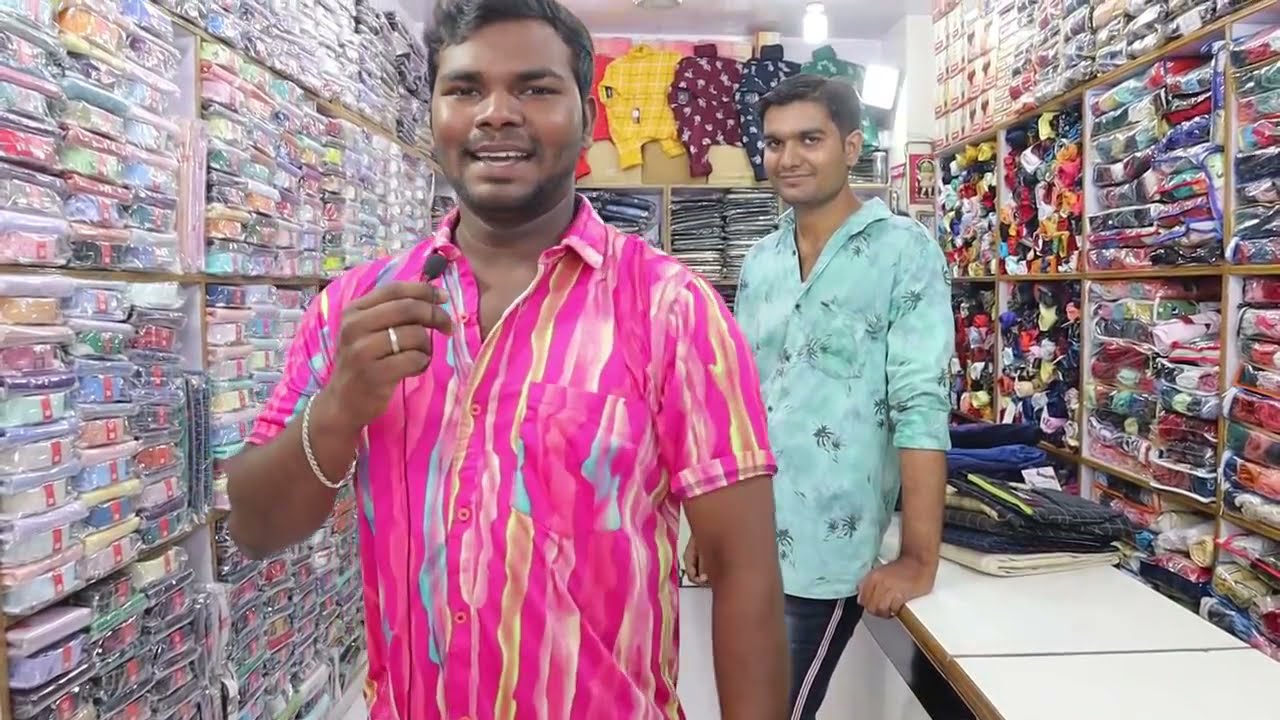This photo captures the lively interior of a small clothing store, possibly situated in a country outside Canada or the United States, with Southeast Asian, likely Indian, characteristics. The store is lined with shelves filled with neatly stacked dress shirts in plastic packaging, and the back wall showcases a variety of shirts pinned up for display. The narrow shop is brightly lit, adding a vibrant atmosphere.

In the foreground, two young men stand, both smiling and looking directly at the camera. The man on the left is dressed in a vivid pink button-up shirt adorned with yellow and blue wavy stripes running vertically and features a pocket. He sports dark hair, a bracelet on his right wrist, and is holding a small portable microphone. Behind him, leaning against a white table with a wooden edge, is the second man wearing a long-sleeved, possibly Hawaiian-style, blue shirt decorated with palm trees. His sleeves are rolled up, and he is dressed in pants with a stripe down the leg. The scene is set against a backdrop of assorted clothing items, with dress shirts on the left, infant clothes in the back, and what appear to be blankets and yarn on the right.